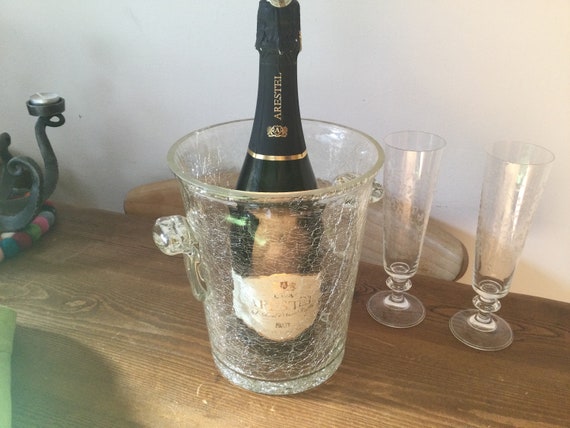A captivating photograph captures an unopened green champagne bottle, labeled "Aristel," elegantly resting inside a uniquely designed crackled clear glass chilling bucket on a wooden table. The bucket, which mimics the appearance of broken yet intact glass, features two handles on its sides. The champagne bottle is adorned with a black top label, a white front label, and gold banding and motifs. Accompanying this setting are two tall, cylindrical champagne flutes next to the bucket, each bearing a similar crackled glass design. To the left of the bucket, a scale and a wrought iron ornamental decoration add to the scene. The background reveals a white wall, while a wooden chair sits in the foreground, contributing to the warm and welcoming atmosphere.